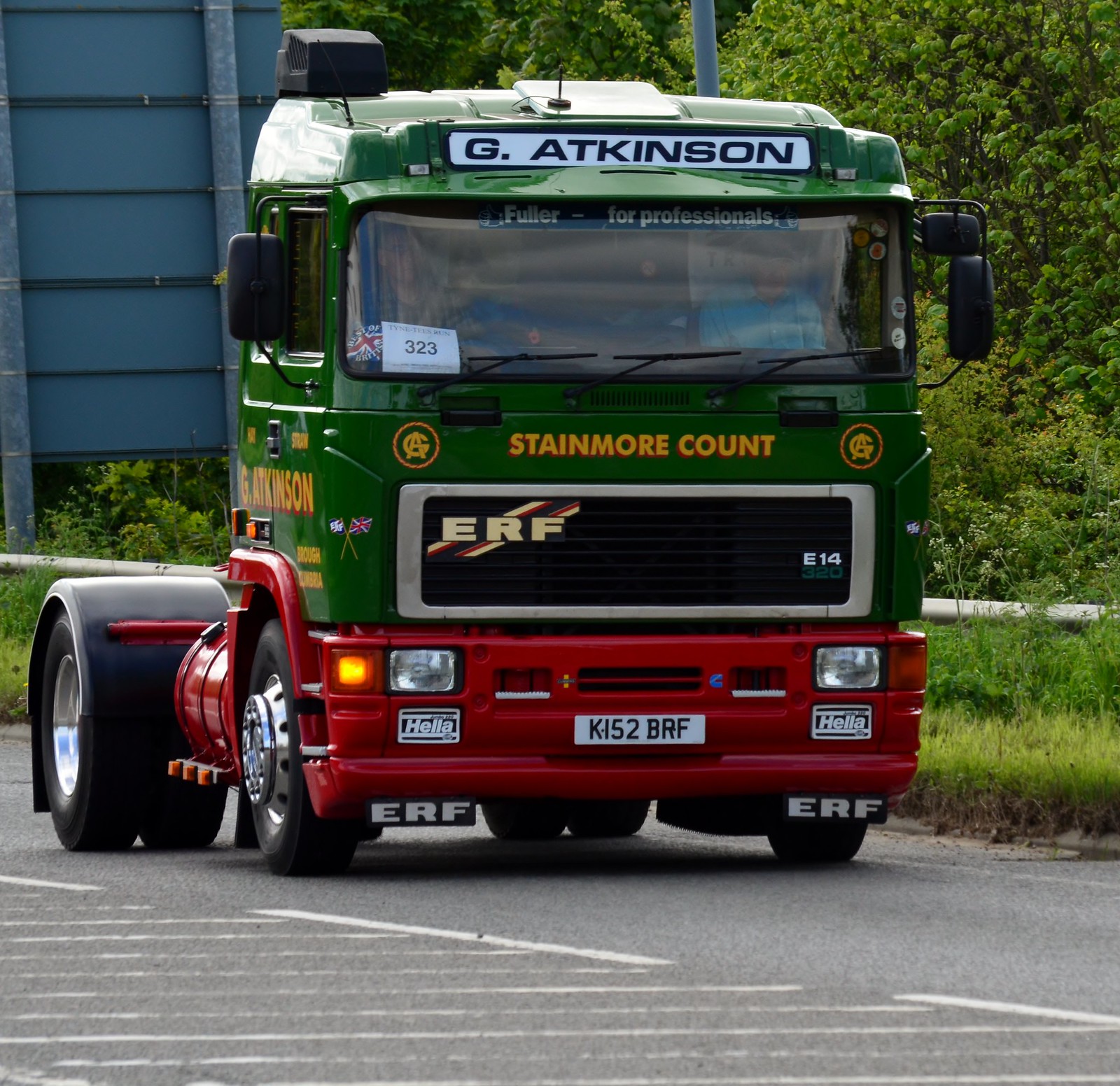This outdoor image features the front of a flatbed truck. The cab of the truck is painted green, while the bumper is red. Above the windshield, there's a white rectangular sign with dark lettering that reads "G Atkinson." Below the windshield, the green section of the cab has yellow text that says "Stainmore Count." The truck's black grill has the letters "ERF" on the top left. The license plate, located on the red bumper, is white with black numbers and letters reading "K152BRF." The cab's side mirrors are black, and the driver, who appears to be wearing a blue shirt, is partially visible through the windshield. A sheet of paper with the number "323" is also visible inside the windshield. Surrounding the truck, there is grass, some trees, and what appears to be a blue shed or road sign in the background, and it is currently parked on pavement.